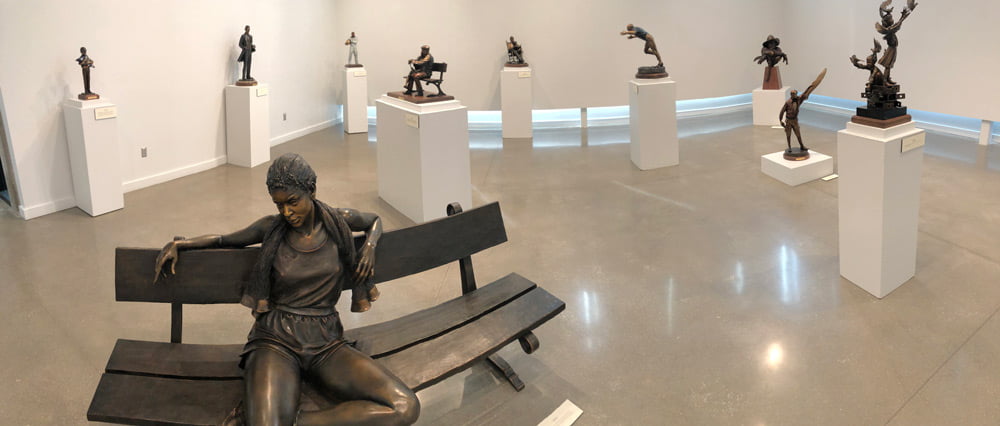The photograph captures a sculpture display within a museum setting. In the background, a series of white display cubes of varying heights showcase an assortment of nine bronze statues. These statues depict a variety of human figures and animals, meticulously arranged against a pristine white wall. The floor beneath them shines with a tan, marble-like finish, adding a touch of elegance to the room.

Dominating the left lower portion of the image is a striking, large bronze sculpture of a park-style bench. Seated on this bench is a woman, sculpted in exquisite detail. She is depicted with her arms casually draped over the backrest, suggesting a moment of relaxation. The woman is adorned in a tank top and running shorts, with a towel hanging around her neck, implying she has paused mid-run to rest and catch her breath. This serene and lifelike portrayal contrasts beautifully with the formal arrangement of the statues in the background, creating a dynamic and engaging scene.